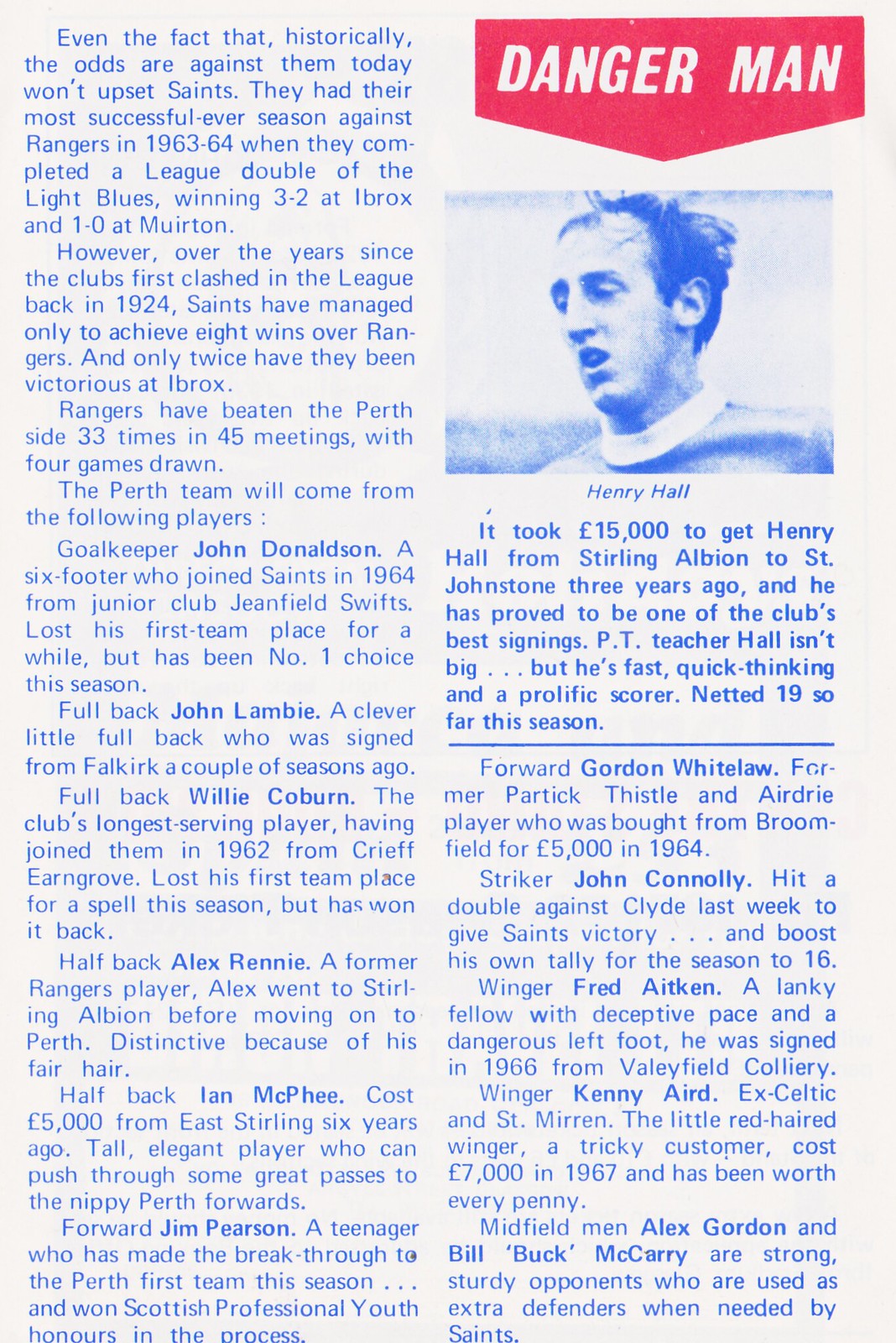The image depicts a slightly yellowed scan of a vintage magazine article portraying a soccer or football theme. The article is printed in blue ink and consists of two columns of text. The left column fully occupies the page, while the right column begins just beneath a picture situated at the top right corner. This picture is a close-up shot of a man's face, identified as Henry Hale by a caption below it. The man appears to be wearing a sport-style shirt and the image has a blue tinge, rendering it virtually colorless aside from shades of blue.

A large red arrow labeled "Danger Man" in white italic bold lettering points down to Henry Hale's image, indicating his significance. The narrative of the article includes historical references to a football league, discussing events such as Saints' notable league double victories against Rangers in the 1963-64 season. This detailed article not only profiles Henry Hale but also delves into the history and achievements of the football league, providing context and background on various historical events and performances.